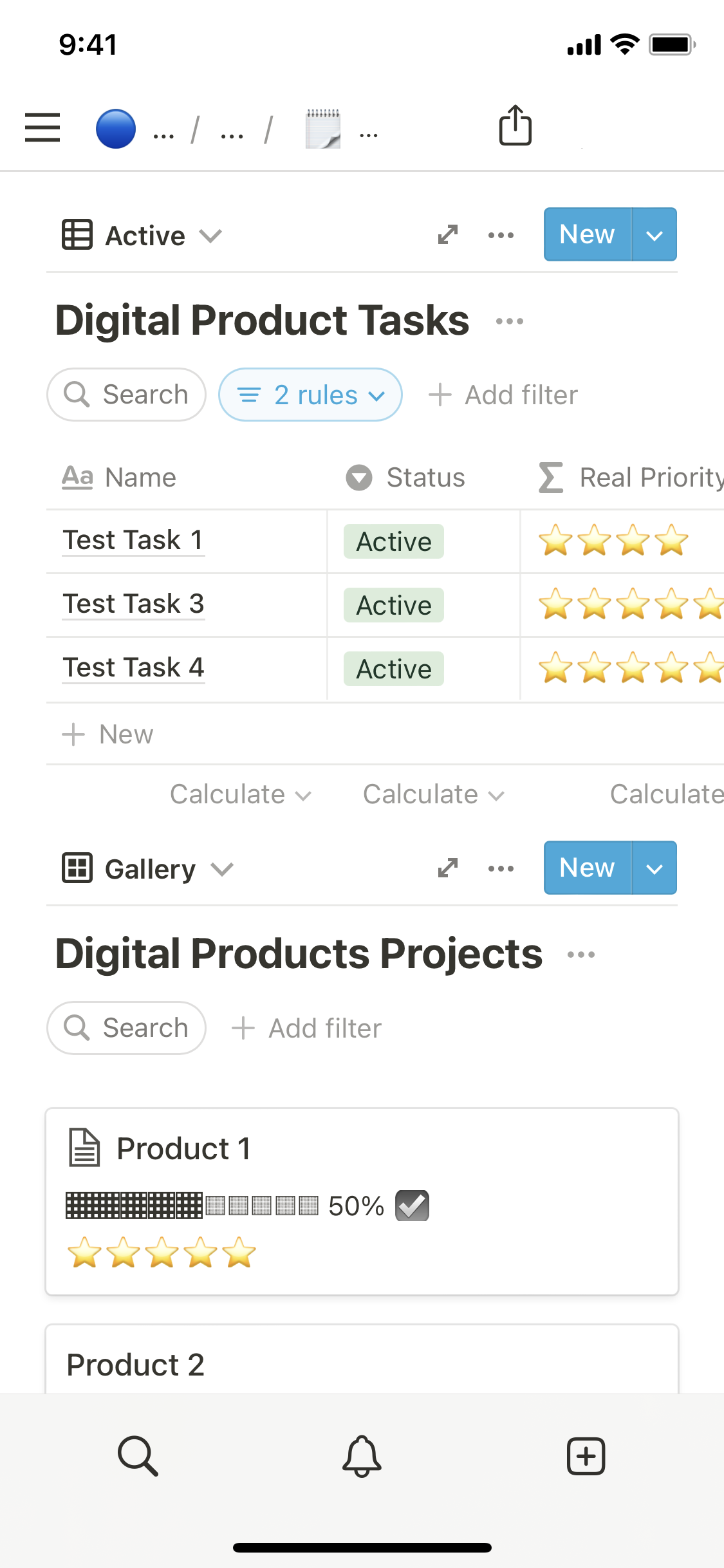The image displays a mobile phone interface featuring various icons, text, and menu options. 

At the top of the screen, the time is displayed as "9:41". To the left of the time is an unidentified symbol, while to the right are indicators showing cellular signal strength, Wi-Fi connectivity, and a fully charged battery.

Below this, there is a navigation bar with several icons: 
- Three horizontal lines stacked vertically (possibly a menu).
- A blue circle containing three dots and a slash.
- An icon resembling a calendar.
- Three more dots.
- An upload icon.

Next, there's a line reading "Active" accompanied by an arrow pointing downward, alongside an unclear line drawing. To the right of this is a double-ended diagonal arrow followed by three dots and a blue rectangle labeled "NEW" in white letters.

Beneath this section, text reads "Digital Products Task" in black. Two ovals are present here, one labeled "Search" and the other "Two Rules." Additionally, there's a "+ Add Filter" option.

The main content area features a table divided into three primary columns:
1. **AA Name**
    - Contains entries: Test Task One, Test Task Three, Test Task Four.
2. **Status**
    - Contains three rectangles, each labeled "Active."
3. **Real Priority**
    - Contains a heading showing a Greek letter (possibly eta or xi), and three rows below it with yellow stars: four stars, five stars, and five stars.

Further down, the interface includes sections labeled "Calculate," "Gallery," and "Digital Products Projects." The "Digital Products Projects" section features another "Search" oval, a "+ Add Filter" option, "Product One" with a "50%" progress indicator and five stars, followed by "Product Two."

Against a bluish-gray background at the bottom are icons for a magnifying glass (search), a bell (notifications), and a plus in a square (add new).